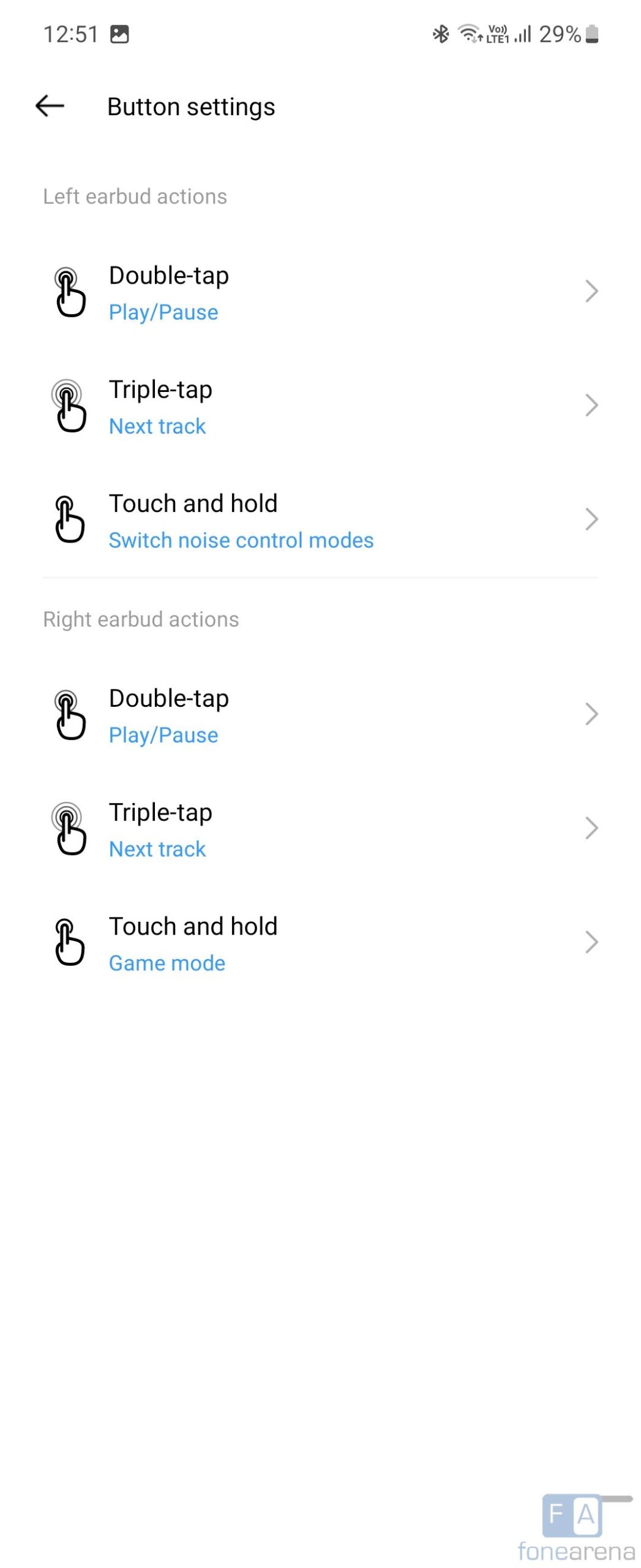The image depicts a screenshot taken from an Android phone. In the top-left corner, the time is displayed as 12:51, accompanied by an icon resembling the symbol seen when a screenshot is captured. The battery level, shown in the top-right corner, is at 29%. The title "Button settings" is prominently displayed in the upper-left section of the page. Below, a list of six options appears, organized in two groups: three for the left earbud and three for the right earbud. These settings are likely for a Bluetooth headset, offering various button functionalities such as double-tap, triple-tap, and touch-and-hold features. The background of the page is white, providing a clean and simple interface.